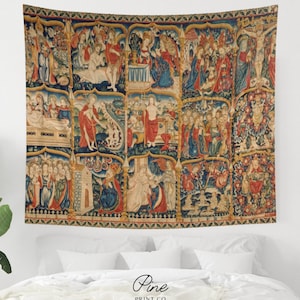The image appears to be a close-up of a bedroom featuring a predominantly white bed with a white duvet cover, two large white pillows, and three smaller white pillows stacked on top. Above the bed's white headboard, a large tapestry hangs on the white wall. This tapestry, reminiscent of a medieval rug, appears to tell a story through 15 small squares arranged in three rows of five. Each square contains intricate images that seem to depict scenes of royalty and possibly religious or medieval events, though the details are somewhat blurry. The tapestry incorporates a color palette of red, brown, blue, and green. To the left of the bed, a green plant with a few leaves visible suggests the presence of an end table. At the bottom of the tapestry, there is a black print that reads "Pine Print Co."